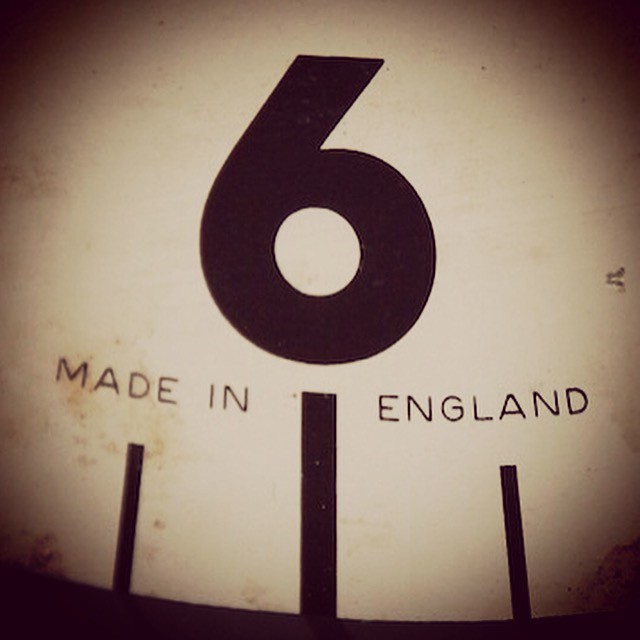This close-up image features a vintage gauge with a distinct black frame. The gauge's face is primarily white, exhibiting signs of age and wear. Centered prominently is a large black numeral six, slightly faded, indicating its central role in the gauge's measurement. Surrounding the main numeral, a thick, black horizontal line runs through the center, flanked by two smaller black lines—one on each side.

Above the horizontal line, the word "MAIDEN" is visible, while "ENGLAND" is positioned below, suggesting the gauge's origin. The white background of the face shows some discoloration and rust around the edges, indicating exposure to environmental elements over time. Shadows cast from a light source add depth to the image, and subtle scratches and marks, including a notable indentation to the right of the six, further tell tales of the gauge’s prolonged use.

The close-up perspective highlights the rounded, circular shape of the gauge, resembling a segment where the number six typically rests at the bottom center. The intricate details of aging, such as the wear on the numeral and the slight fading of the black markings, contribute to the gauge's historical charm.